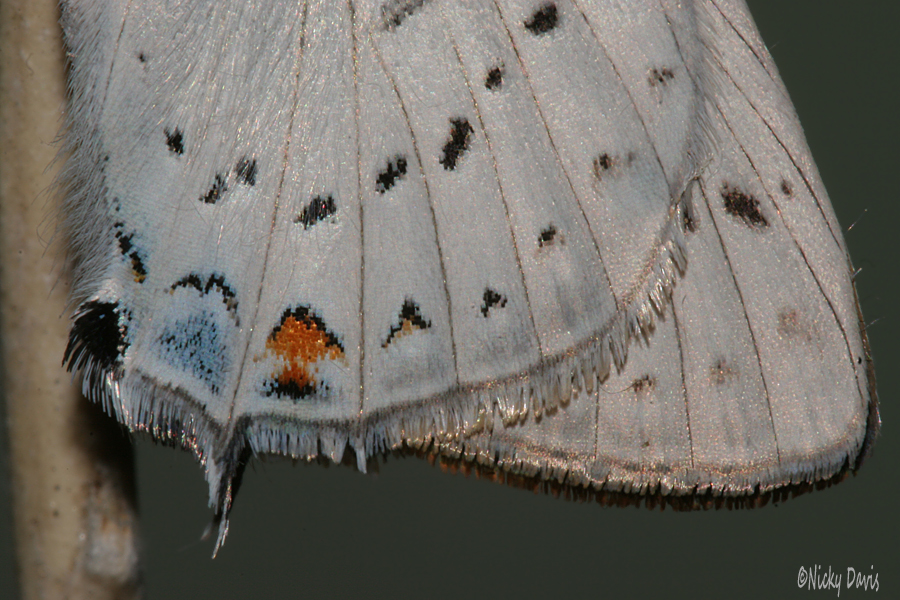This is a very close-up image capturing the intricate details of a butterfly's wings, focusing on their lower sections. The butterfly's body is not visible, emphasizing the delicate pattern of the wings. The background is a solid dark gray, and in the lower right corner, the photograph is credited to Nikki Davis, written in white cursive. On the left side of the image, there is a faint presence of a light tan-brown tree branch.

The wings, which dominate the frame, display a silvery white color with vertical brown lines and rows of uniformly patterned spots. The spots near the middle are predominantly black, while those towards the bottom exhibit vibrant hues, including orange and blue, bordered by black. The wings also feature intricate wavy fringes along their edges, adding to their delicate appearance. The image beautifully captures the texture and color variations, with the left wing prominently visible, overlapping the partially seen right wing.